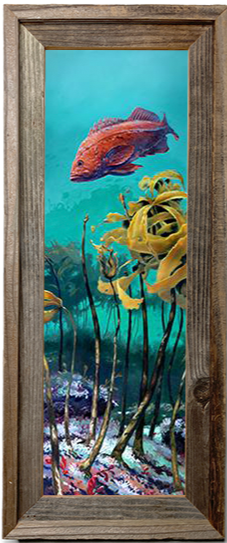This photograph captures a vertically oriented, narrow, rectangular painting encased in a rough, homemade-looking wooden frame. The dark pine wood frame is wide, with a two-tiered design where the inner tier slopes inward toward the painting, and features a noticeable knot hole toward the right side. The wood varies in color, displaying brownish-gray hues and darker tones on the lower half, accentuating its rustic appeal.

The painting itself depicts a vivid underwater scene rendered in a turquoise blue-green background. Dominating the scene is a vibrant red fish swimming gracefully. Beneath the fish, long narrow stalks rise from the multicolored ocean floor, which is adorned with hues of blues, pinks, and reds, and scattered with underwater vegetation. Among the plants are delicate yellow flowers with long, stringy petals that stretch upward near the fish, adding to the lush, aquatic ambiance. It's a piece of art so detailed and striking that it could easily be featured in a catalog or on a website for purchase.